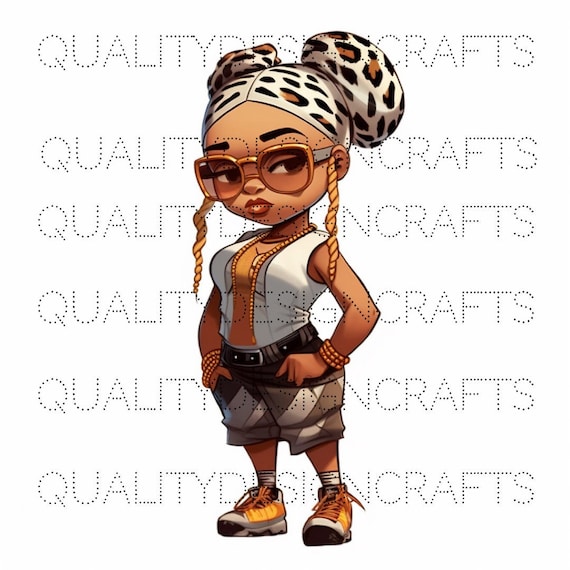The clip art features a stylish black woman with caramel-colored skin. She has her hair tucked under a zebra-print hat, with golden strands or braids spilling out from either side. The hat seems to gather her hair into buns. Her face is framed by trendy gold or metallic glasses, and she appears to be pursing her lips, giving her an air of attitude.

Her outfit includes a white sleeveless shirt under a vest with gold detailing in the center, paired with tan and brown cuffed shorts. She cinches the ensemble with a dark brown belt featuring a silver buckle. On her feet, she sports yellow tennis shoes with orange laces, white tips, and grey accents, accompanied by crew socks. Accessorizing further, she wears brown beads on both her wrists.

The background is transparent, emphasizing the character, and overlaying the image are six lines of text that read "quality design crafts" in small dotted letters, serving as a sort of watermark or signature for the illustration.